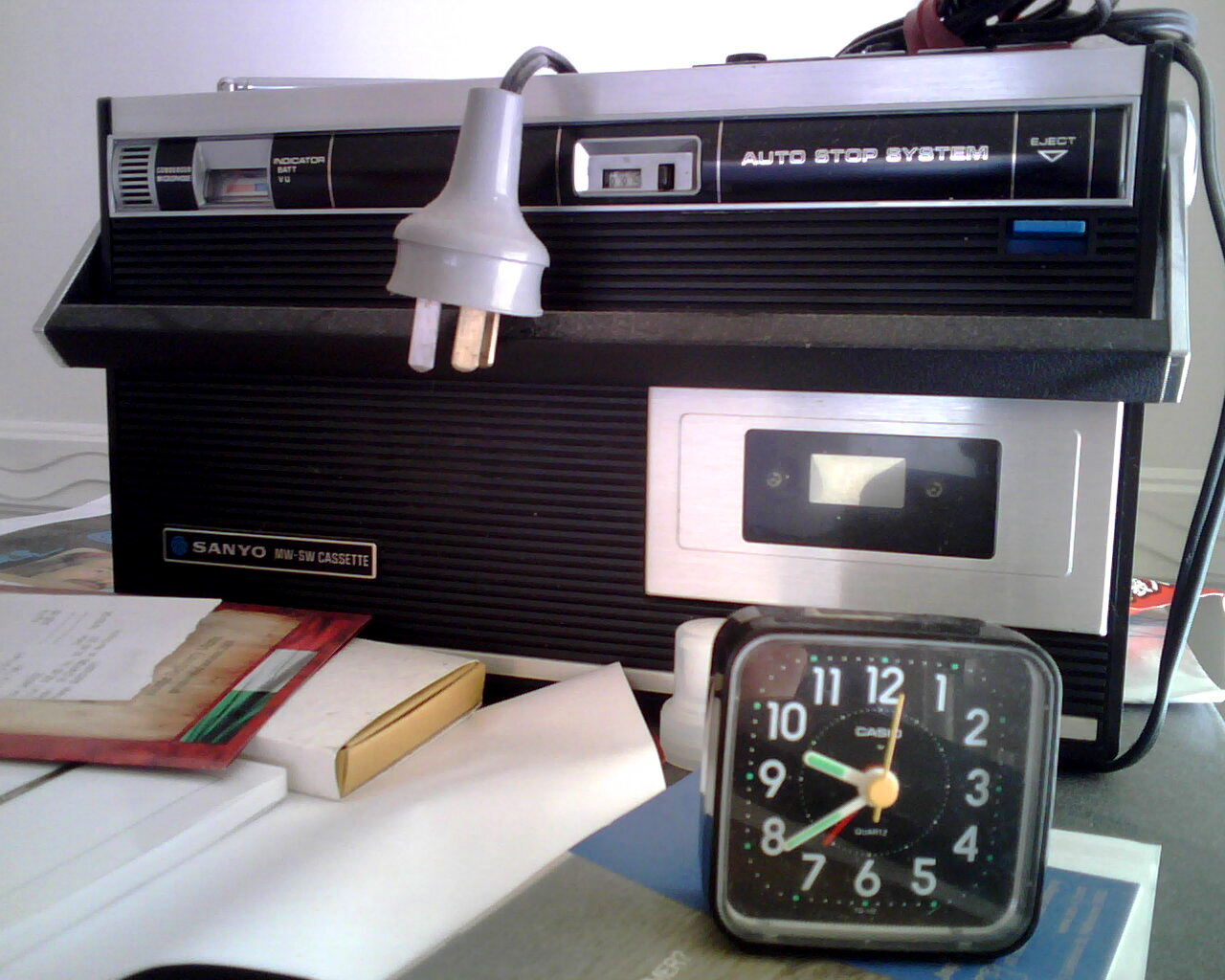In this color photograph, a small, old-fashioned cassette boombox is prominently featured. The boombox is black and silver, with the brand name "Sanyo" visible in the bottom left corner. The tape deck, which is lighter silver in color, is situated on the right side with a clear window revealing the two small tape spinners. Above the tape deck, the words "Auto Stop System" are inscribed in silver, and nearby is a blue eject button marked with a downward arrow. A thick cord with a gray plug drapes over the boombox, and one of the plug pins is illuminated, giving it a golden appearance. The top of the boombox features a battery meter labeled "Indicator Battery" and some dials on the upper left. The long black handle of the boombox is pushed down over the top, collecting noticeable dust.

In front of the boombox is a small square alarm clock with black casing and white numerals. Its glow-in-the-dark green hour and minute hands point to around 9:40, while it also has smaller yellow and red hands. Both items rest on a small gray table cluttered with books, tapes, papers, and possibly a clipboard with a red top. The backdrop, strewn with various objects, adds to the sense of a cozy, nostalgic space filled with tangible memories.